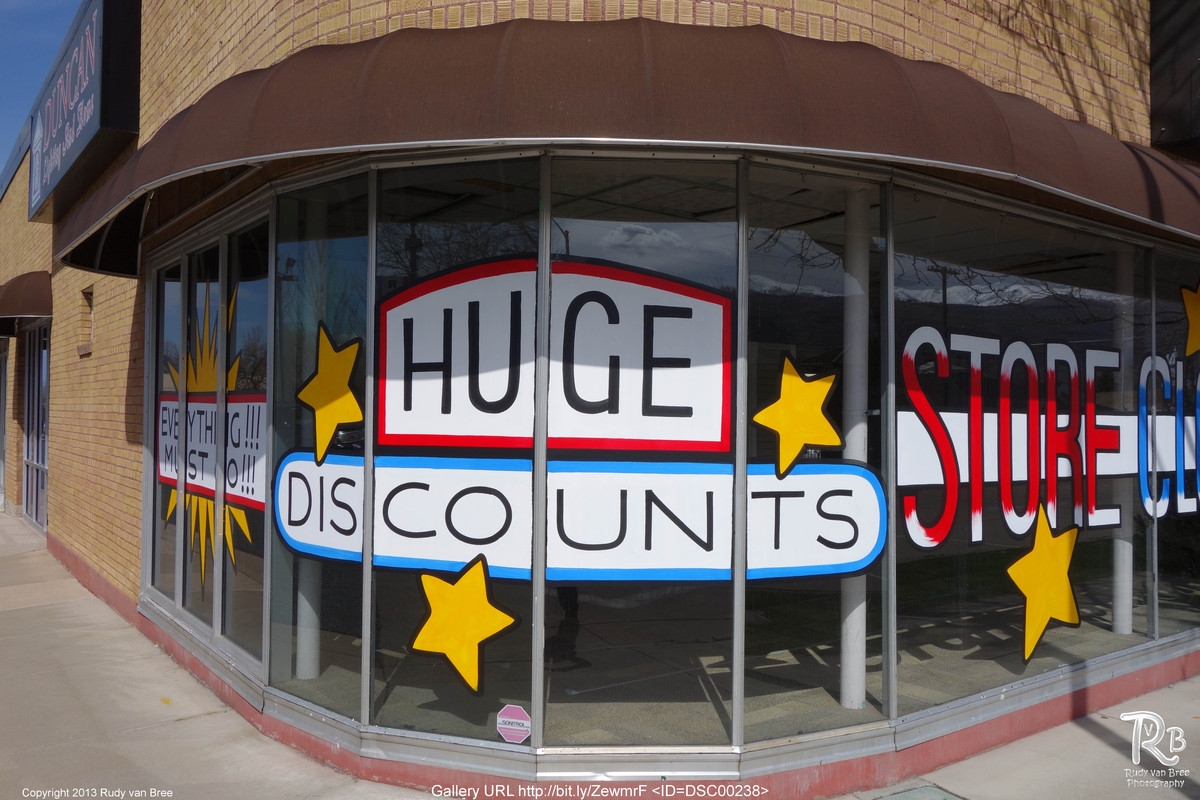The photograph captures a close-up view of the corner of a unique, intersection-building with an intriguing design. The building, situated at what could be a complex intersection, features a curved store front on the first floor, characterized by expansive windows and a brown canopy overhead. The prominent signage on the rounded front showcases the words "HUGE DISCOUNTS" in a striking design: the phrase is printed in black letters on a white background, with the word "HUGE" outlined in red and "DISCOUNTS" edged in light blue. Four gold stars accompany the text, adding a touch of flair.

Additionally, on the left window, as the storefront curves around, there's a sign proclaiming "EVERYTHING MUST" with a large gold starburst behind it, implying an urgent message. On the right side, another sign displays the enormous word "STORE" in bold red letters with white tips, and partly visible below it is "CL," suggesting the word "CLOSING."

Above these windows, the building's facade is composed of tan bricks, enhancing its classic architectural appeal.